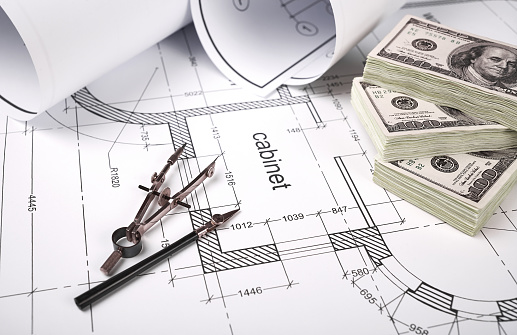In this detailed, color photograph with a landscape orientation, a neatly arranged desk hosts a set of scaled floor plan drawings, rendered in black ink on a white background. The central area of the floor plan prominently features the word "Cabinet," surrounded by various dimensions and architectural details such as walls and a curved window section. Atop the left part of the blueprint lies two silver and black drafting tools: a protractor and what appears to be a fountain pen, lying at an angle. Near the top left and center of the image, a couple of rolled-up blueprint pages add depth to the scene. Dominating the right side are three staggered stacks of $100 bills, fanning out with the central stack pointing left, the top stack pointing to the top right, and the bottom stack pointing to the bottom center. The bills are neatly arranged but are cropped by the right edge of the image. The scene captures a realistic and meticulously organized workspace.